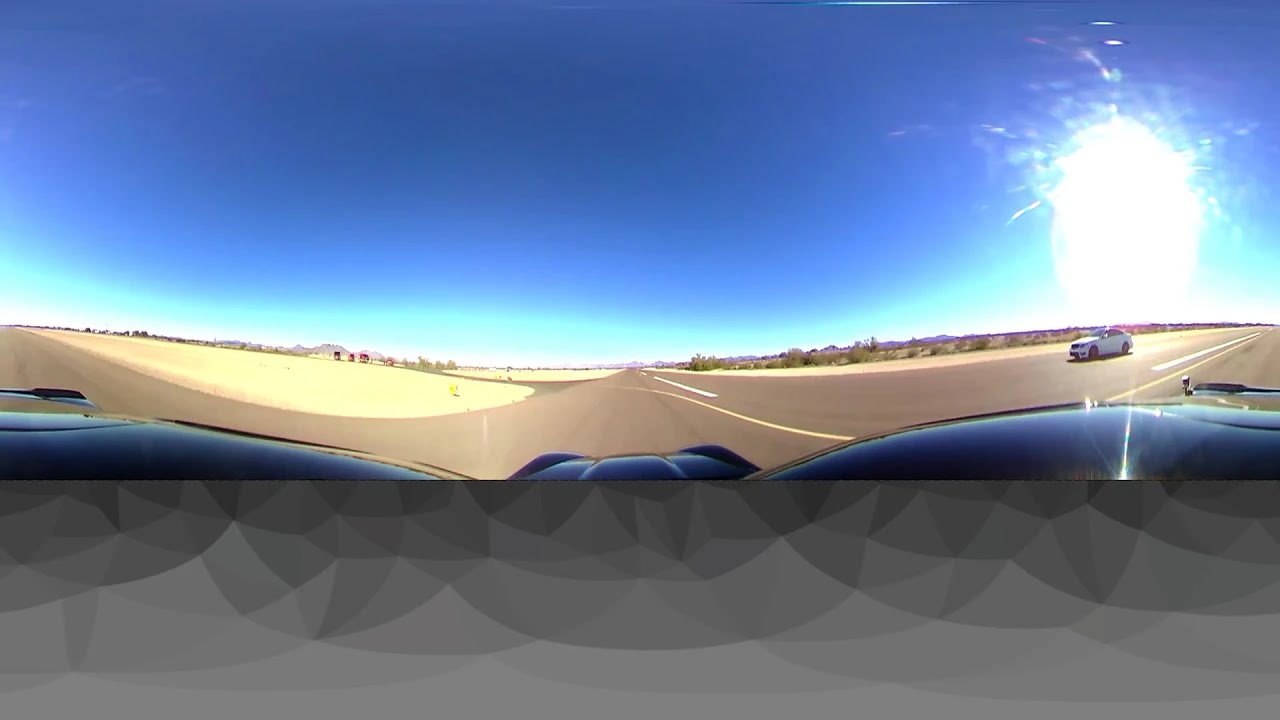The image depicts a wide-angle shot taken from inside a moving car on a straight roadway, likely in a desert setting. The vantage point suggests the use of a GoPro or similar camera mounted on the hood of the black, shiny car, which reveals a sloped hood. The road, which runs horizontally through the center of the shot, features clean white lines and appears well-maintained. On the right side of the image, a white four-door sedan is seen approaching from the opposite direction. 

The surroundings are predominantly barren with expansive stretches of sand on both sides, though some sparse vegetation is visible to the right. A prominent mountain range spans the background to the left, characterized by its brown hues and minimal green, mostly confined to the mountain's peak. The sky above is a clear blue with almost no clouds, giving the impression of a bright, sunny day. The sun itself is positioned in the upper-right corner, casting a bright light over the scene. The overall setting evokes a mid-day desert atmosphere, complete with the distinctive multi-textured gray tones of the landscape.